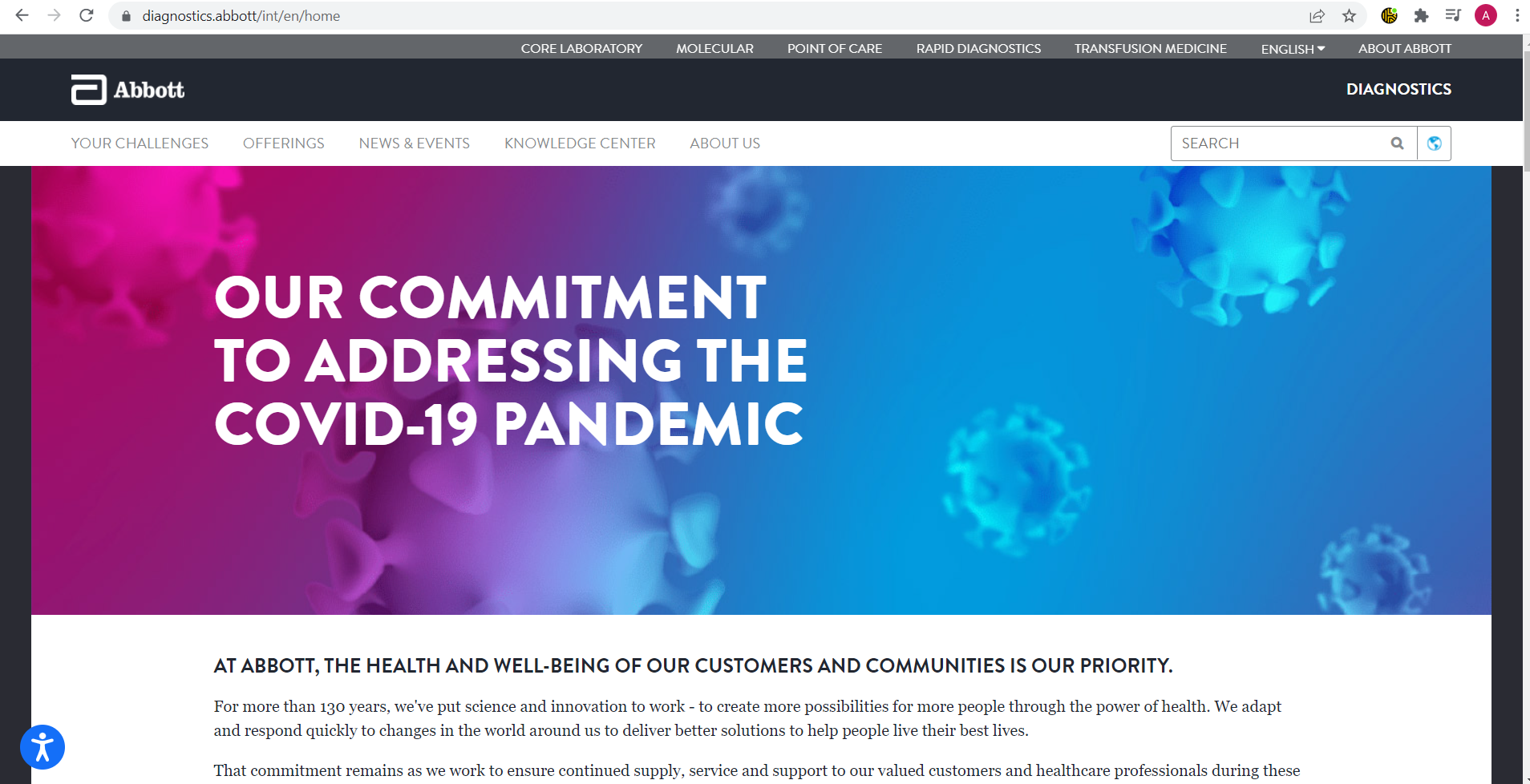The image depicts a webpage with the URL "diagnostics.about/int/int/home." The webpage features several navigational links, including "Core Laboratory," "Molecular," "Point of Care," "Rapid Diagnostics," "Transfusion Medicine," "English," "About," "Your Challenges," "Offerings," "News and Events," "Knowledge Center," "About Us," "Search," and "Our Commitments to Addressing the COVID-19 Pandemic." A prominent section of the page emphasizes the company's dedication to the health and well-being of its customers and communities, stating that for over 130 years, they have leveraged science and innovation to create new possibilities through the power of health. The company prides itself on its ability to adapt and respond quickly to global changes, aiming to provide better solutions to help people live their best lives. This commitment is reiterated as the company ensures the continued supply, service, and support for their valued customers and healthcare professionals during challenging times.